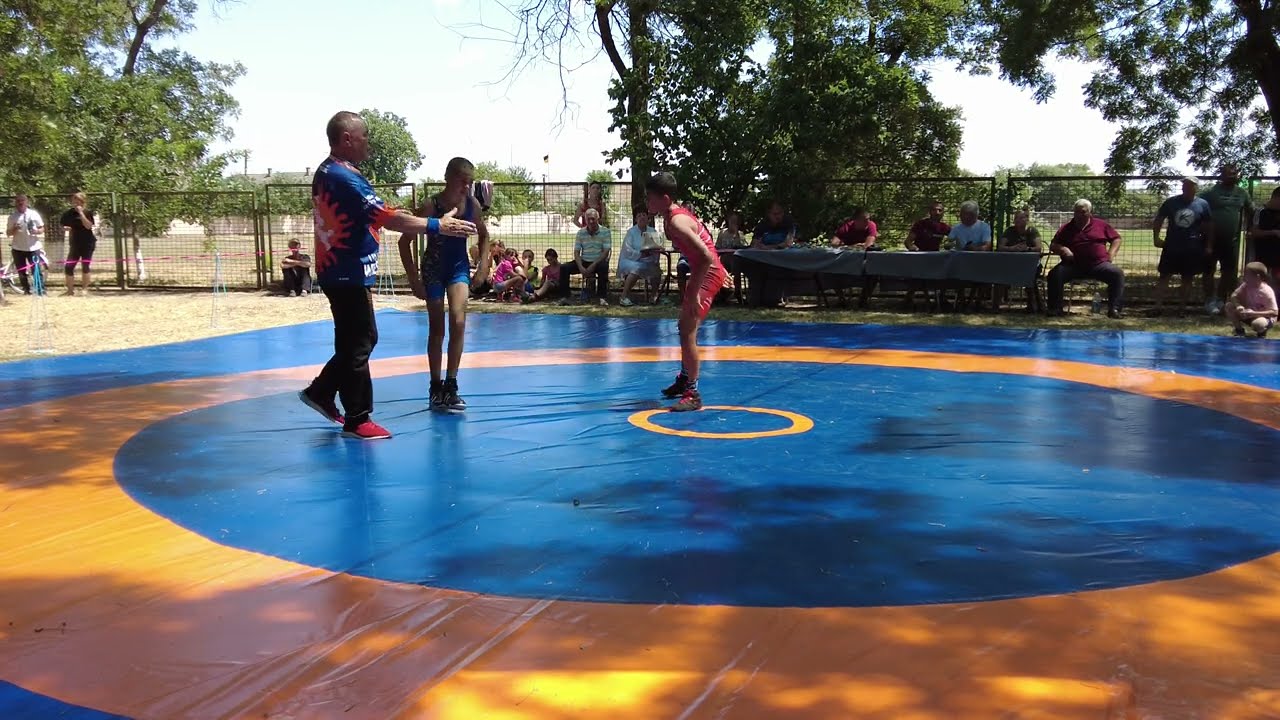This vibrant color photograph, in landscape orientation, captures an action-packed outdoor wrestling match set in a park. Central to the image is a large wrestling mat, distinguished by its layered design: a bright blue circular center, encompassed by an orange ring with another blue circle encircling it, and finally a smaller orange circle at its core. On the mat, two young boys stand poised for competition, dressed in traditional wrestling singlets. The boy in the blue outfit stands centrally facing the camera, while the boy in the red outfit faces him from a few feet away. To the left, a referee clad in a colorful tie-dye shirt, black pants, and red sneakers, extends his arm as if signaling points or initiating a handshake. The setting is bustling with activity; behind the wrestlers, a crowd gathers, comprising spectators seated at a table, individuals leaning on a fence, and others simply enjoying the park ambiance. Trees and a fence frame the background, adding a serene touch to this energetic scene. The detailed composition effectively captures the intensity of the match and the communal atmosphere of a lively park setting.